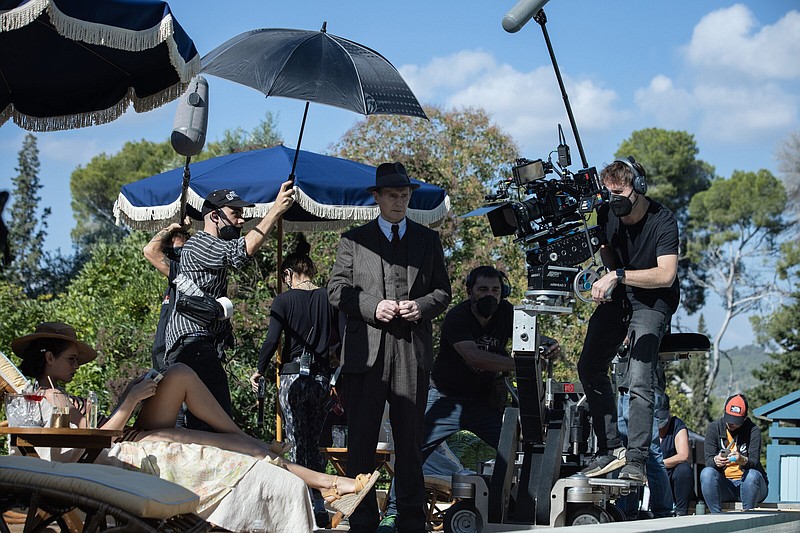In a detailed behind-the-scenes photo from a film set, an actor, who bears a resemblance to Kevin Kline, stands thoughtfully at the center, dressed in a dark, three-piece suit and a matching hat. His hands are clasped together, suggesting deep contemplation. To his left, a woman lounging in a bikini under a large parasol by the pool is engrossed in a book, which might actually be her phone. The setting appears to be the backyard of a house. Surrounding them is a bustling film crew: multiple camera operators are positioned up close, catching every nuance, and a technician stands holding an umbrella to control the shot's lighting. The detailed organization reveals the intricate efforts involved in creating a movie scene.